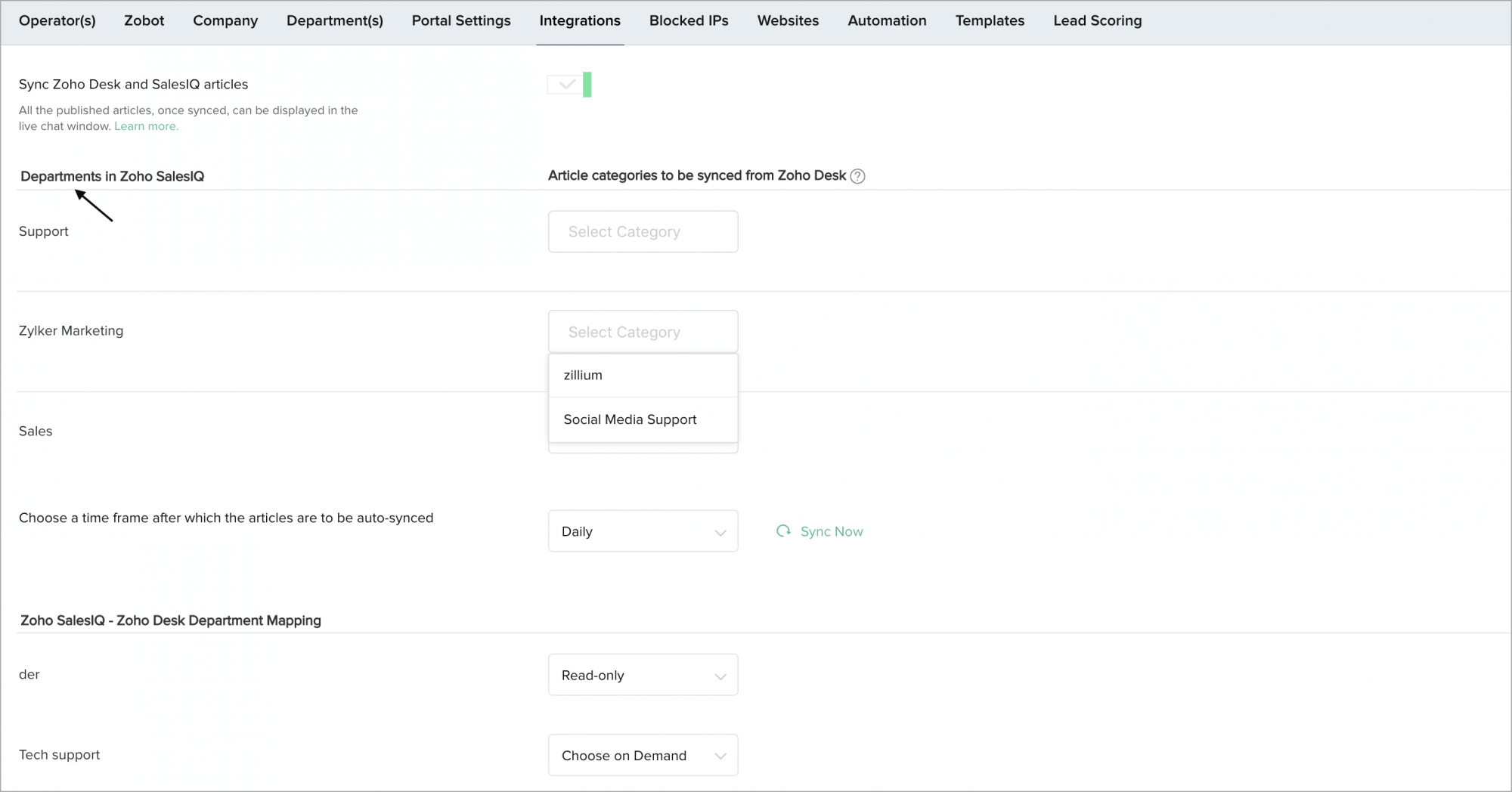The screenshot displays a comprehensive view of a sales department website. At the top, a horizontal gray bar spans the width of the screen and contains menu items: "Operators," "Zobot Company," "Departments," "Portal Settings," "Integrations" (which is underlined to indicate selection), "Locked IPs," "Websites," "Automation Templates," and "Lead Scoring." 

Beneath this bar, there are options titled "Sync Zoho Desk" and "SalesIQ Articles" with the subtitle "All the portals will sync." A live chat window is prominently displayed alongside a "Learn More" link highlighted in green, with a checkmark next to it, indicating activation.

Further down, the interface shows navigation for "Departments," specifically within "Zoho SalesIQ," with sections such as "Support" indicated by an arrow for ease of navigation. The "Article Categories" section features drop-down options to "Sync Zoho Desk" and a category selection option that currently has no specific category selected. 

One drop-down menu includes options like "Zilker Marketing" and "Zillium or Social Media Support," while another context menu partially obscures "Sales."

Additionally, there is an option to "Choose a timeframe which articles are to auto-sync daily" accompanied by a light green "Sync Now" button. In the lower section, "Zoho SalesIQ" and "Zoho Desk Department Mapping" are bolded, with "DER" marked as read-only and "Tech Support" showing a selectable on-demand option. The overall interface appears to be part of a larger sales support program designed for syncing and managing support articles and department mappings in Zoho.